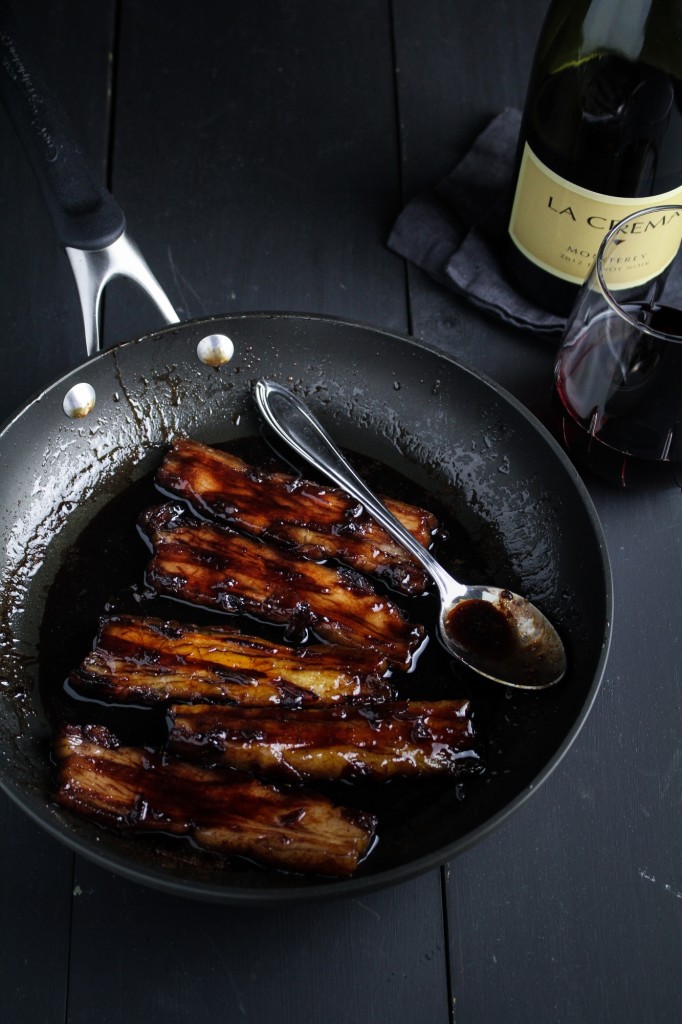The image is a detailed close-up, top-down photograph capturing a black table with a black frying pan, which features silver bolts and a silver attachment connecting to a black handle. The frying pan contains approximately five spare ribs smothered in a thick, dark barbecue sauce with charred bits. A silver spoon lies across the last rib, still holding some of the dark sauce. To the right, there is a partially filled glass of red wine and behind it, a green wine bottle with a tan label reading "La Crema," sitting on a piece of black cloth. The entire scene highlights the rich, dark tones of the barbecue ribs alongside the elegance of the accompanying wine.